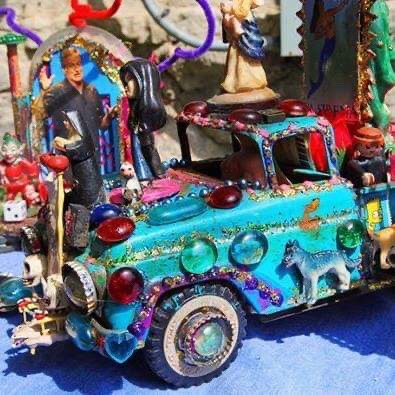The image depicts a lively scene centered around a highly adorned miniature model truck, painted in a rich teal color. The truck is an older style with numerous decorative elements attached, creating a festive atmosphere reminiscent of a parade or celebration. Gems, bottle caps, and other trinkets embellish it, including bottle caps with inserted gems serving as headlights and hubcaps. In the truck bed, a Lego figure and other small figurines are visible, adding to the cluttered and vibrant composition.

A four-legged animal, possibly a stylized wolf, is among the many adornments, along with a small toy man waving, evoking a sense of joyful activity. The detailed truck sits in front of a background where a woman with long black hair, clad in a blue garment, stands, almost as if overseeing the scene. To the left, a figure resembling a gnome straddles the boundary, contributing to the whimsical nature of the tableau. Additionally, various colorful decorations like dice, red and purple accents, and a possible Buddha statue complete this eclectic and richly detailed spectacle.